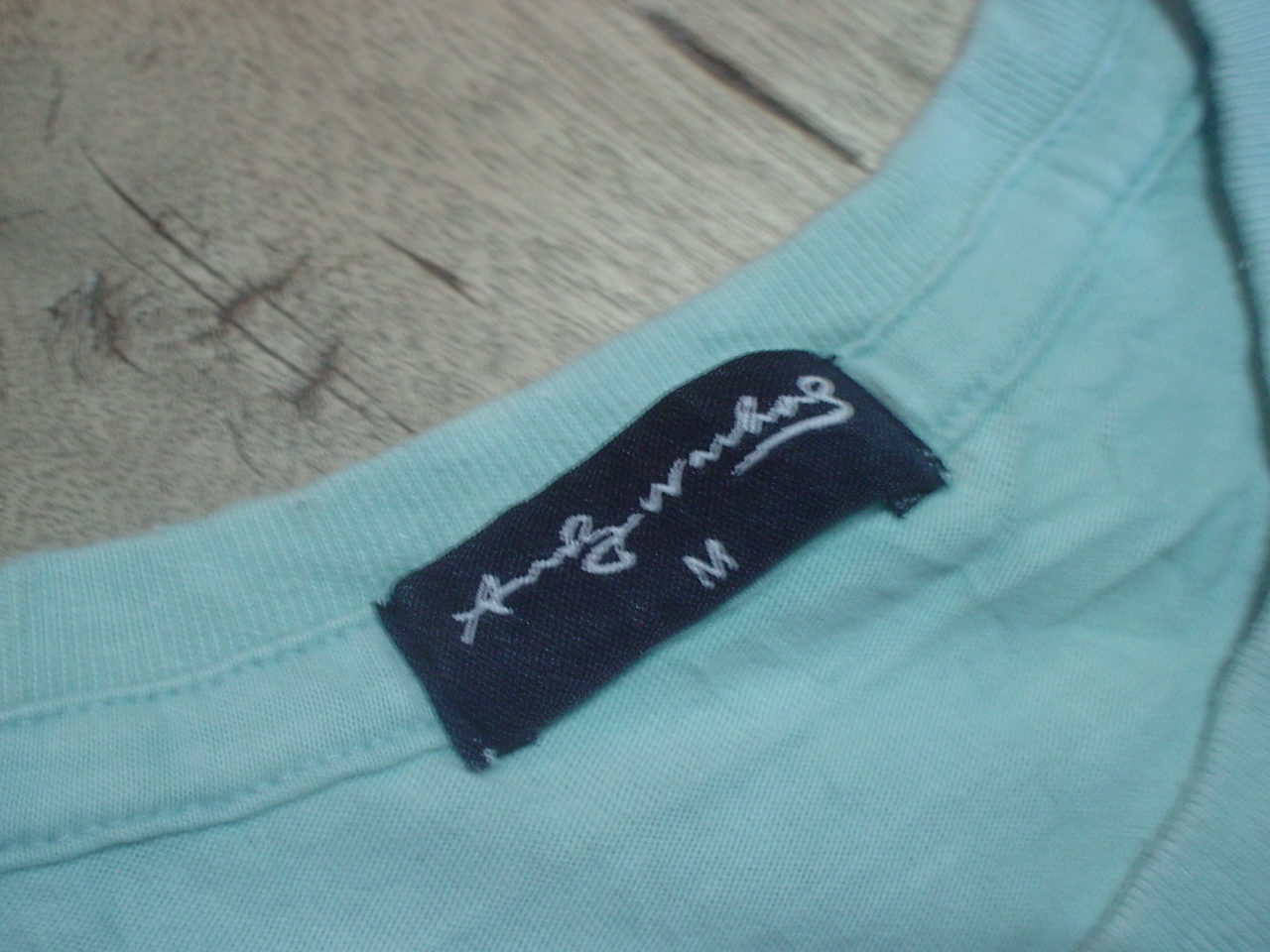The image showcases a close-up view of the back neckline of a teal green garment, which could be either a shirt or a sweater, as the specific type is indiscernible from the photograph. The focus of the image is on a black, rectangular tag sewn into the fabric, displaying white text. The brand name on the tag is partially visible, with potential initials that start with an "A" or a "W," followed by a handwritten style script. The tag clearly indicates the garment is a size medium. The garment is laid out on a white, wooden desk that has a slight grayish hue, although it is not the focal point of the image. The composition emphasizes the details of the tag and the garment’s color and texture.